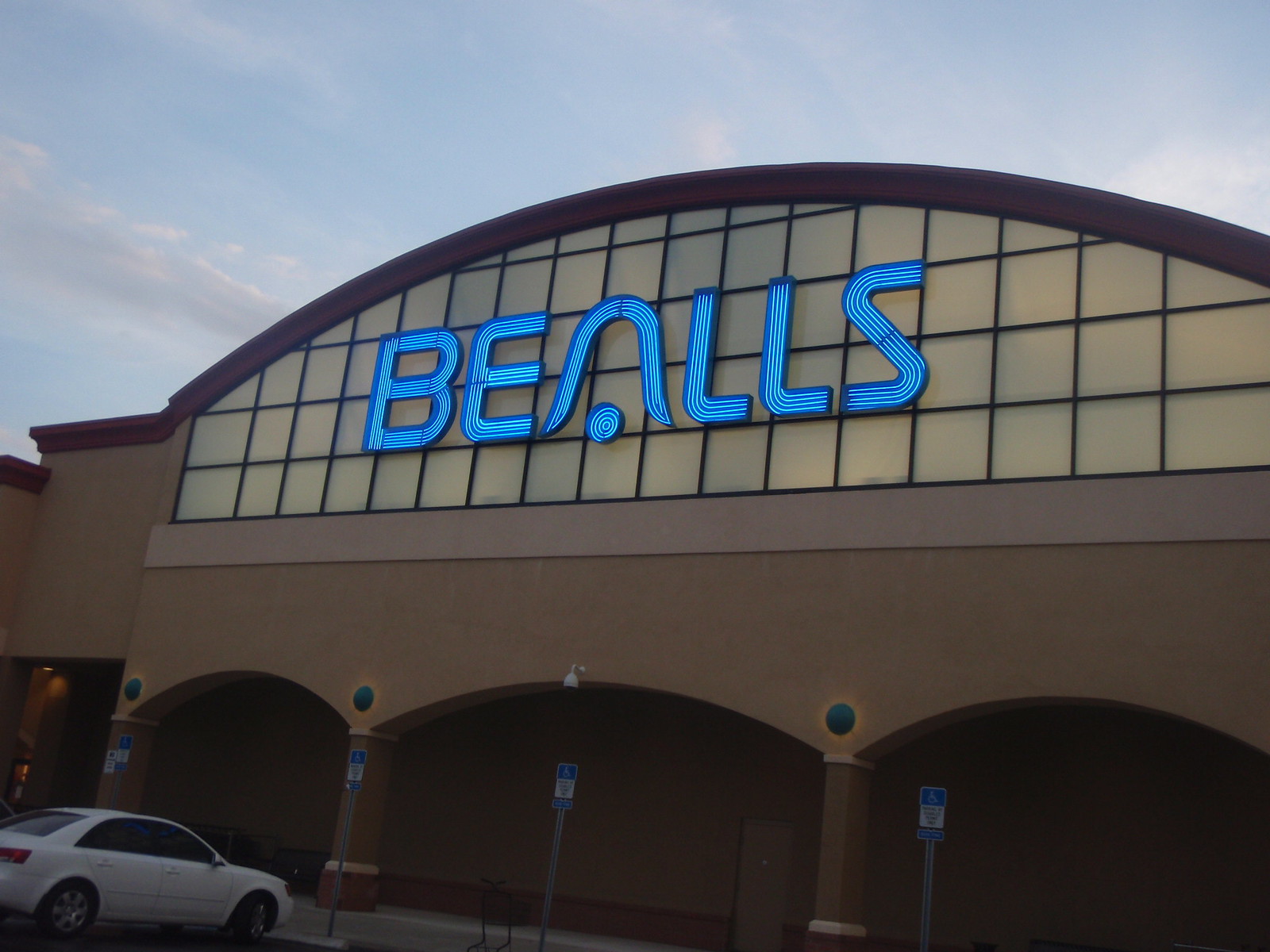The image captures an outdoor scene in a parking lot of a large retail establishment named "Bealls" (B-E-A-L-L-S), often mispronounced as "Beals." The photograph is taken from a first-person point of view, slightly tilted upwards to capture the building’s facade. The building features an arched top with a distinctive grid motif and scalloped edges at the bottom, creating a structured appearance. Prominently displayed on the facade are blue, illuminated letters forming the store name, with the letter "A" stylized to resemble a bell with a curved top and a dot in the center. Below the storefront, the image shows four handicap parking spaces, identifiable by the blue signage atop poles indicating disability parking. One white car is parked in the leftmost handicap spot. The scene is set against a cream or beige background with black lines, under a clear blue sky with scattered clouds.